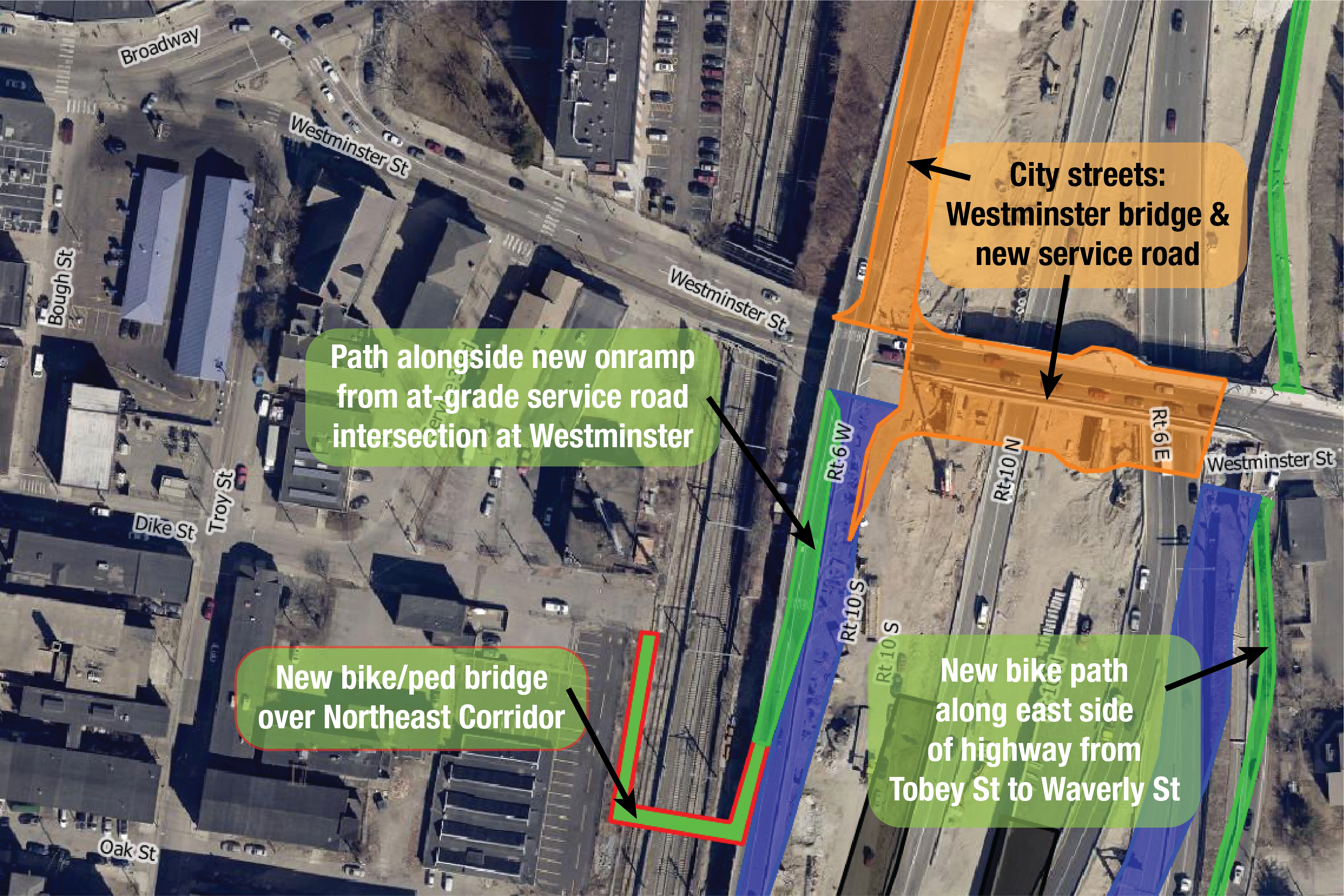This image presents an aerial view, reminiscent of a Google Maps screenshot, capturing a cityscape from above. The prominent feature is a large bridge, labeled as Westminster Bridge, which is highlighted in an orange text box reading "City Streets, Westminster Bridge, and New Service Road." Numerous roads weave through the city, including Westminster Street, Troy Street, and Broadway, all clearly marked with their names in black text outlined in white. The visualization includes multiple construction and planning highlights. Green sections with white text identify future infrastructure projects, such as a “New Bike Path along East Side of Highway from Toby Street to Waverly Street,” and “New Bike, Ped Bridge, over Northeast Corridor.” Another green text box shows a “Path alongside New On-Ramp from At-Grade Service Road intersection at Westminster.” Cars are visible both parked in lots and moving along the roads, while the tops of buildings form a patchwork against the streets. The map, supplemented with arrows and color-coded sections in green, blue, and orange, details planned additions and modifications to the urban layout, providing a comprehensive overview of current and future developments from a high vantage point.